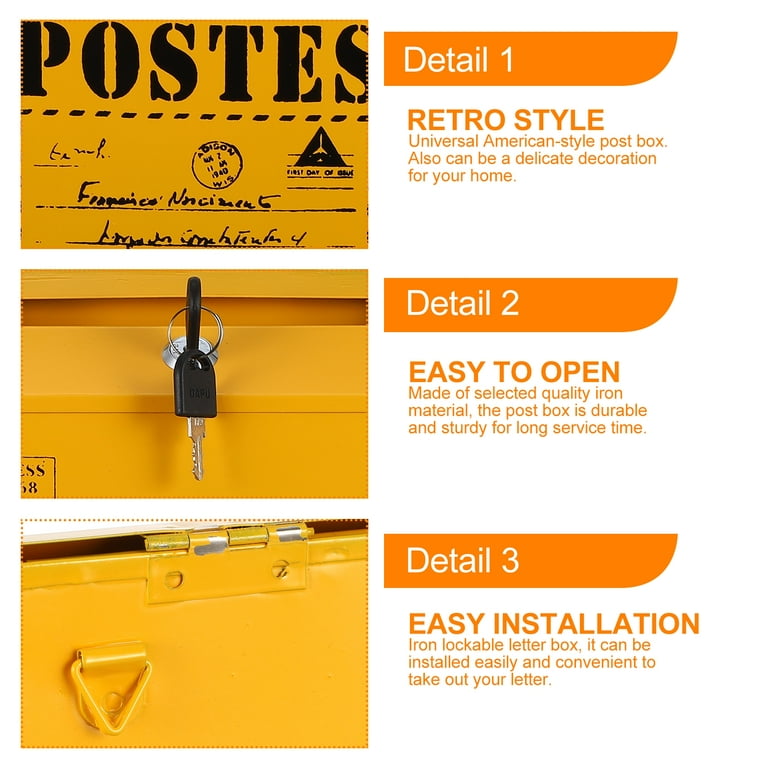The image provides detailed instructions and advertisements for a Universal American Style Post Box, divided into three segments. The left-hand side features three stacked pictures. At the top, "Detail 1" showcases a letter labeled "Posties," describing the retro style of the post box, emphasizing that it can also serve as a delicate home decoration. The middle image, "Detail 2," features a key hanging from a hook, highlighting the easy-to-open functionality and the high-quality iron material, which ensures durability and long service time. The bottom segment, "Detail 3," shows a yellow lockable letter box with a triangular handle, boasting easy installation and convenient letter retrieval. Collectively, these images and descriptions serve as a comprehensive template for marketing the key features of the mailbox.